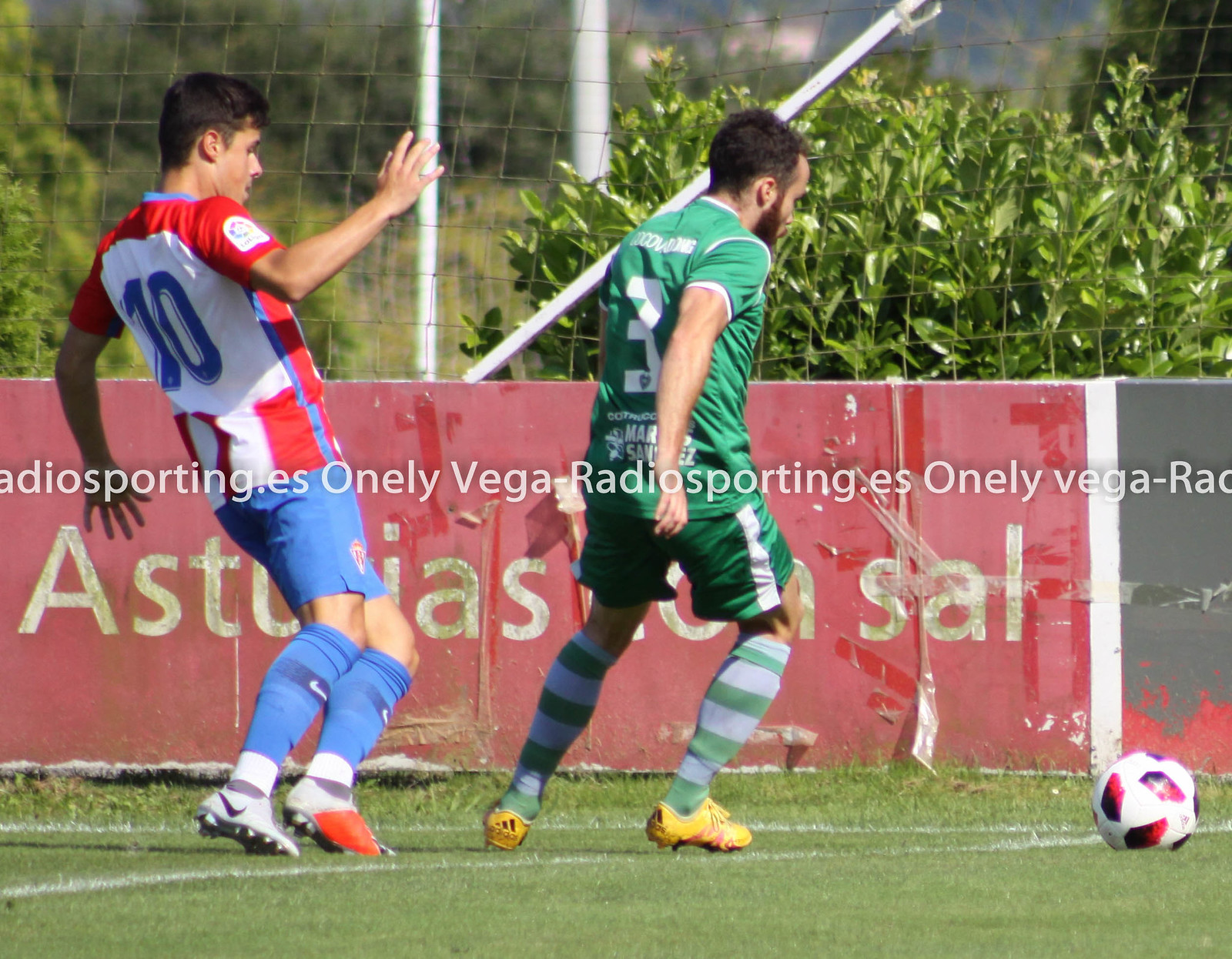This detailed photograph captures a dynamic soccer match between two players on a green grass field marked with white lines. The player on the far left, wearing a distinctive jersey with white backing and red detailing on the shoulders and sides, is bearing the number 10. He is outfitted in blue shorts, blue socks, and white shoes with an orange patch on one. Centrally positioned is the opposing player, dressed in a green jersey numbered 3, complemented with green shorts featuring white stripes, green and gray socks, and yellow cleats. The action centers around a white soccer ball, intricately detailed with purple, pink, and white, reflecting light in the bottom right corner of the frame.

Behind the players, a weather-beaten red banner with partial text "AST...SAL" can be seen, partially obscured by the athletes. Above this, a horizontal banner stretches across the field, advertising "RadioSporting.es" with repetition indicating "OnlyVega-RadioSporting.es." To the right, lush vegetation contrasts with the metallic silver piping, supporting netting indicative of a goalpost. The atmosphere of the image is vividly brought to life with the textures of the grass, the vibrant colors of the jerseys, and the energetic engagement of the players.